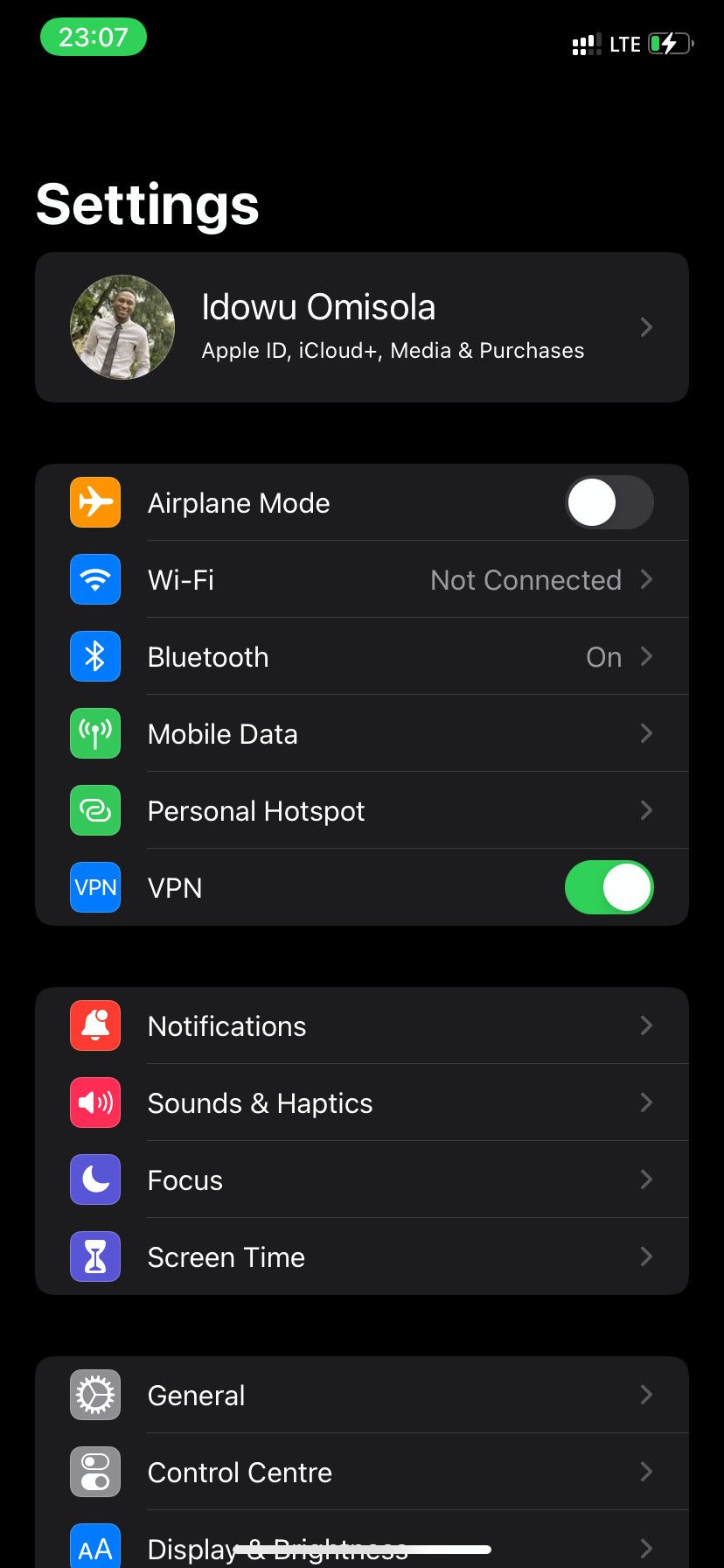Screenshot of an iPhone's Main Settings Page

The image is a screenshot of the main settings page from an iPhone, featuring a black background with neatly organized sections and colorful icons. At the very top, the status bar displays standard icons including battery charge, network strength, and the current time. Below this, the title "Settings" is prominently shown alongside the user's profile picture and name, "Aiduo Omisola", with options for managing Apple ID, iCloud, media, and purchases.

The first visible block of settings includes essential connectivity options such as Airplane Mode, Wi-Fi, Bluetooth, Mobile Data, Personal Hotspot, and VPN, each equipped with toggle switches for quick enablement or disablement.

The subsequent section features settings for Notifications, Sounds & Haptics, Focus, and Screen Time, allowing users to manage how their device communicates with them.

Visible at the bottom of the screenshot are the beginning options of another settings cluster, showcasing General, Control Center, and Display & Brightness. The image clearly indicates that there are more settings available if the user were to scroll further. The familiar layout and icons confirm that the device is an iPhone.